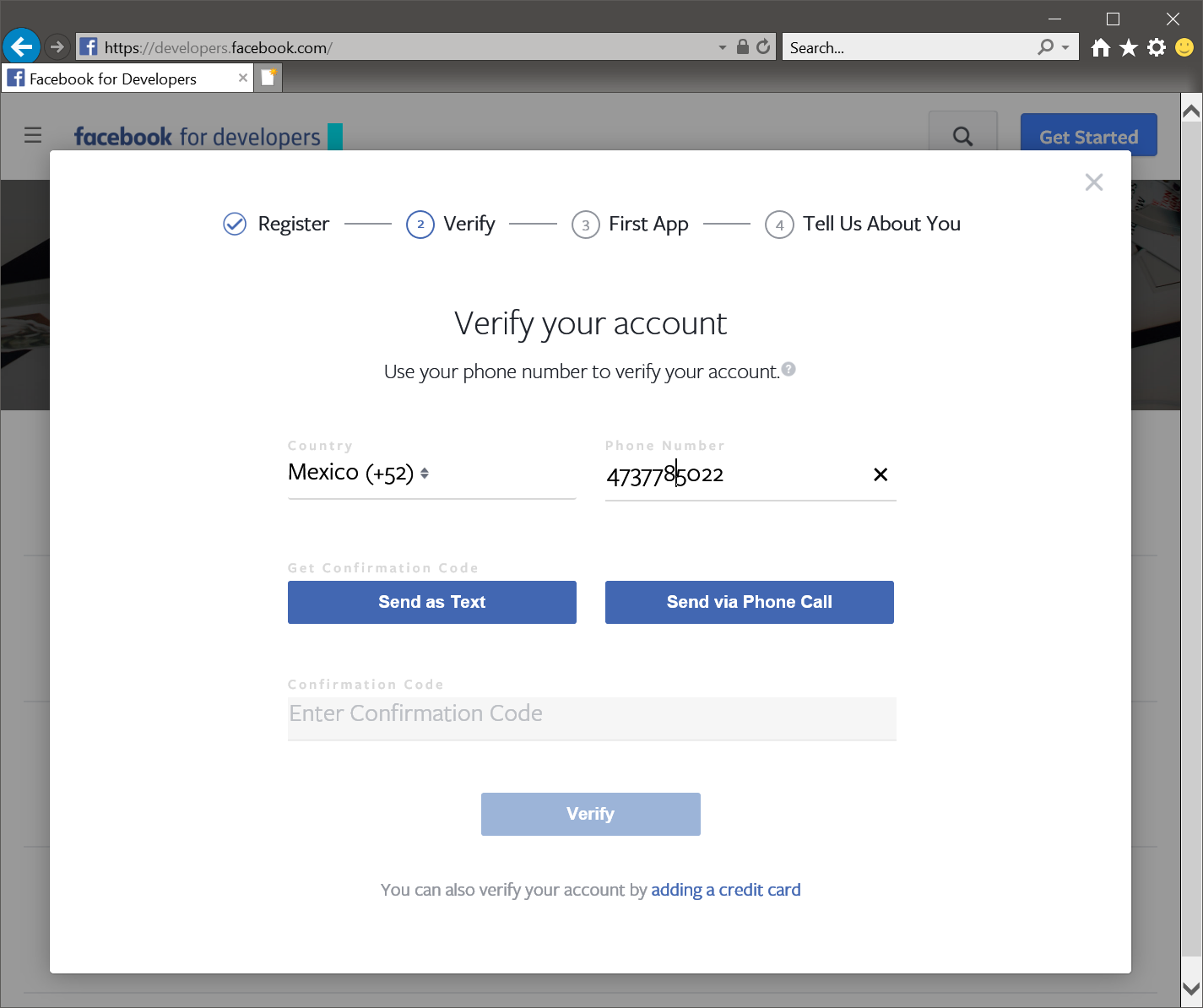This image is a detailed screenshot of the Facebook Developers page, specifically focusing on the account verification process. The URL displayed in the browser's address bar is "https://developers.facebook.com", and prominently on the page in blue text, it reads "Facebook for Developers".

Overlaying this main content is a pop-up window titled "Verify Your Account." This window instructs users to verify their accounts using their phone numbers. The pop-up has a clean white background with black text for clarity. 

Within the pop-up, there is a drop-down menu labeled "Country," where the user has selected Mexico, automatically filling in the country code "+52". Adjacent to this drop-down menu is a field where a phone number is entered; in this case, the number listed is "473-778-5022".

Below the phone number field, there is a section labeled "Get Confirmation Code." Users have two options for receiving their confirmation code, each represented by a blue rectangle with white text: "Send as Text" and "Send via Phone Call."

Beneath these options, there's a field to input the confirmation code once it is received. Following this input field, there is another button labeled "Verify," which users likely click to complete the verification process.